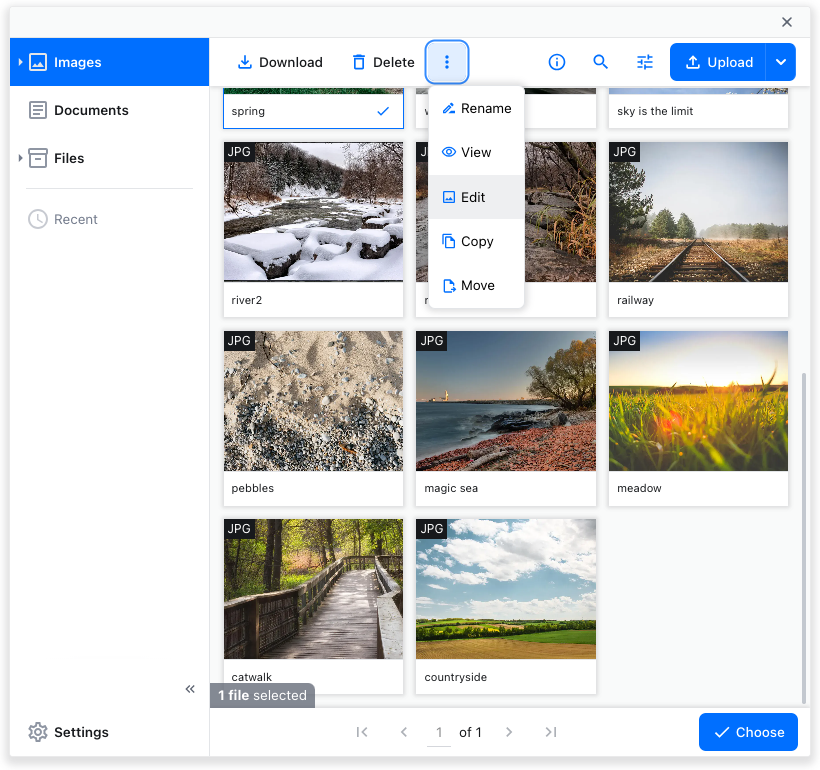Screenshot of a File Management Interface

This screenshot captures a file management interface that allows users to download, delete, and manage images, documents, and other files. Various functionalities are accessible, such as renaming, viewing, editing, copying, and moving files through a drop-down menu. The interface also includes settings and an option to upload files.

The visible files are a collection of picturesque and diverse images:

1. **Icy River**: A serene icy river with ice blocks and visible water flow.
2. **Railroad**: A long shot of an empty railroad extending into a field, framed by a beautiful landscape.
3. **Pebble Beach**: A beach area scattered with pebbles, some partially buried, others exposed.
4. **Magic Sea**: A scenic body of water with pristine sand and pebbles along its shore.
5. **Meadow**: A vibrant meadow with grass glistening under the sunlight.
6. **Catwalk**: A lengthy bridge designed for walking, stretching across a scenic area.
7. **Countryside**: A breathtaking depiction of the countryside, with clear skies, fields, and plains.

These images appear well-suited for use in various projects, such as website templates, documents, or presentations, providing users with an accessible and easy-to-navigate platform for their file management needs.